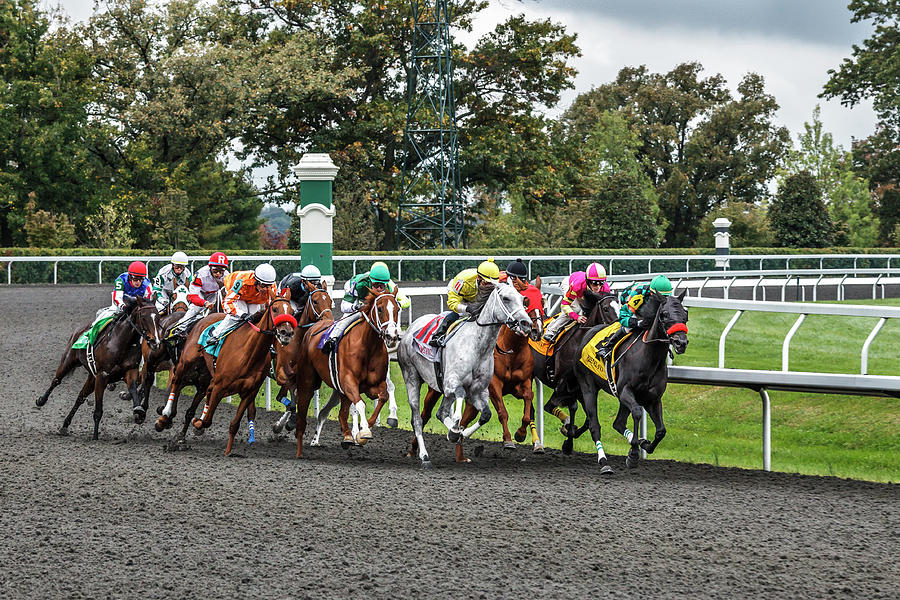The photograph captures a dynamic horse racing scene on a dark grey, curved track featuring approximately 10 horses running closely together. The horses vary in color, including black, brown, and white. Each horse has a rider dressed in distinct, brightly colored uniforms such as yellow, pink, green, orange, blue, and red. One notable detail is a black horse leading the pack, ridden by a jockey in a green helmet, followed closely by a white horse with a rider in a yellow helmet. The right side of the track is bordered by a white fence that encloses a grassy field, while the background showcases a backdrop of trees under an open sky. The scene is further complemented by large green posts with white tops, adding to the vibrant and detailed atmosphere of the race.